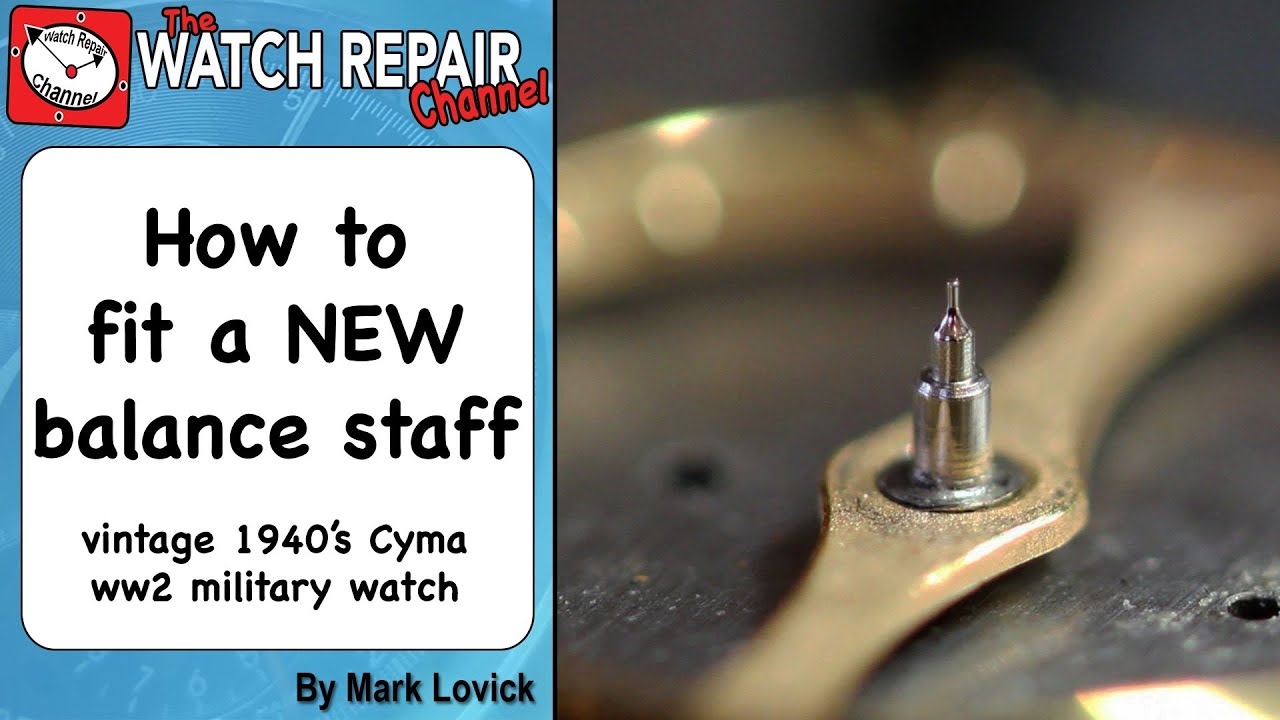The image is a promotional material for a watch repair channel. The left half features a blue background adorned with black text. Prominently, colorful letters spell out, "The Watch Repair Channel." In the upper left corner, there’s a small red square containing the same phrase, and next to it, a partial image of a clock or watch is visible. Below this, the text instructs on "How to Fit a New Balance Staff" for a "Vintage 1940s CYMA WWII Military Watch" by Mark Lubick. The right half of the image displays a close-up view of the intricate inner workings of a watch. The central focus is on a gold screw that secures the watch hands, set against a blurred golden watch face, highlighting the fine details and craftsmanship involved in watch repair.